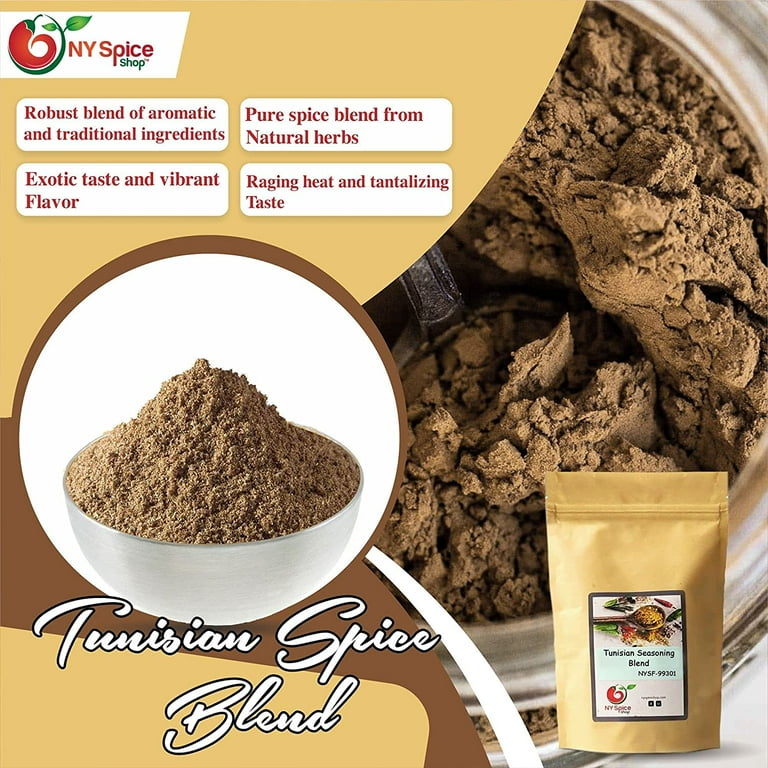The advertisement features the NY Spice Shop's Tunisian Spice Blend. Dominating the top left corner is the shop's vibrant logo, a stylized red chili pepper set against a yellow backdrop, accompanied by the text "NY Spice Shop" in bold red and green lettering. The centerpiece of the ad emphasizes the product's luxurious qualities, with four descriptive phrases: "robust blend of aromatic and traditional ingredients," "pure spice blend from natural herbs," "exotic taste and vibrant flavor," and "raging heat and tantalizing taste." A hero image showcases the spice blend in a white bowl, heaped high with the light brown powder. This is highlighted within a crisp circular frame, with a more extensive backdrop depicting the spice in a container being scooped up. Towards the bottom left, the name "Tunisian Spice Blend" is elegantly written in a cursive font. To the bottom right, a resealable tan-yellow pouch, labeled "Tunisian Seasoning Blend" and featuring the same NY Spice Shop logo, reinforces brand consistency. The overall aesthetic of the advertisement harmonizes tan, brown, and white hues, providing a cohesive and inviting look.